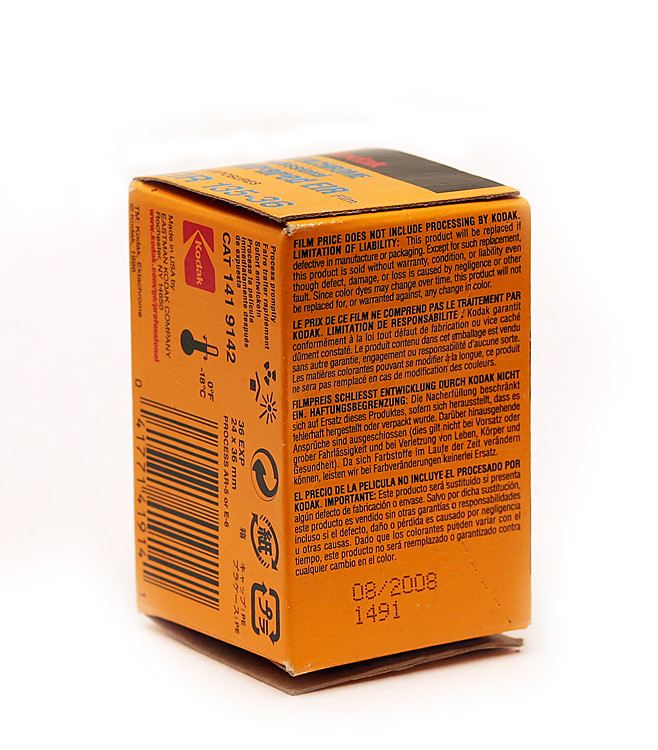This color photograph captures a close-up of the backside of a Kodak film box, prominently showcasing Kodak's iconic yellow packaging. Centered in the frame, the backside reveals a side panel featuring a barcode and the distinctive red Kodak logo. The most visible portion is the back panel, densely covered in very fine print that remains largely illegible. However, a date stamped in the corner stands out, indicating either the expiration date or the date of manufacture as August 2008.